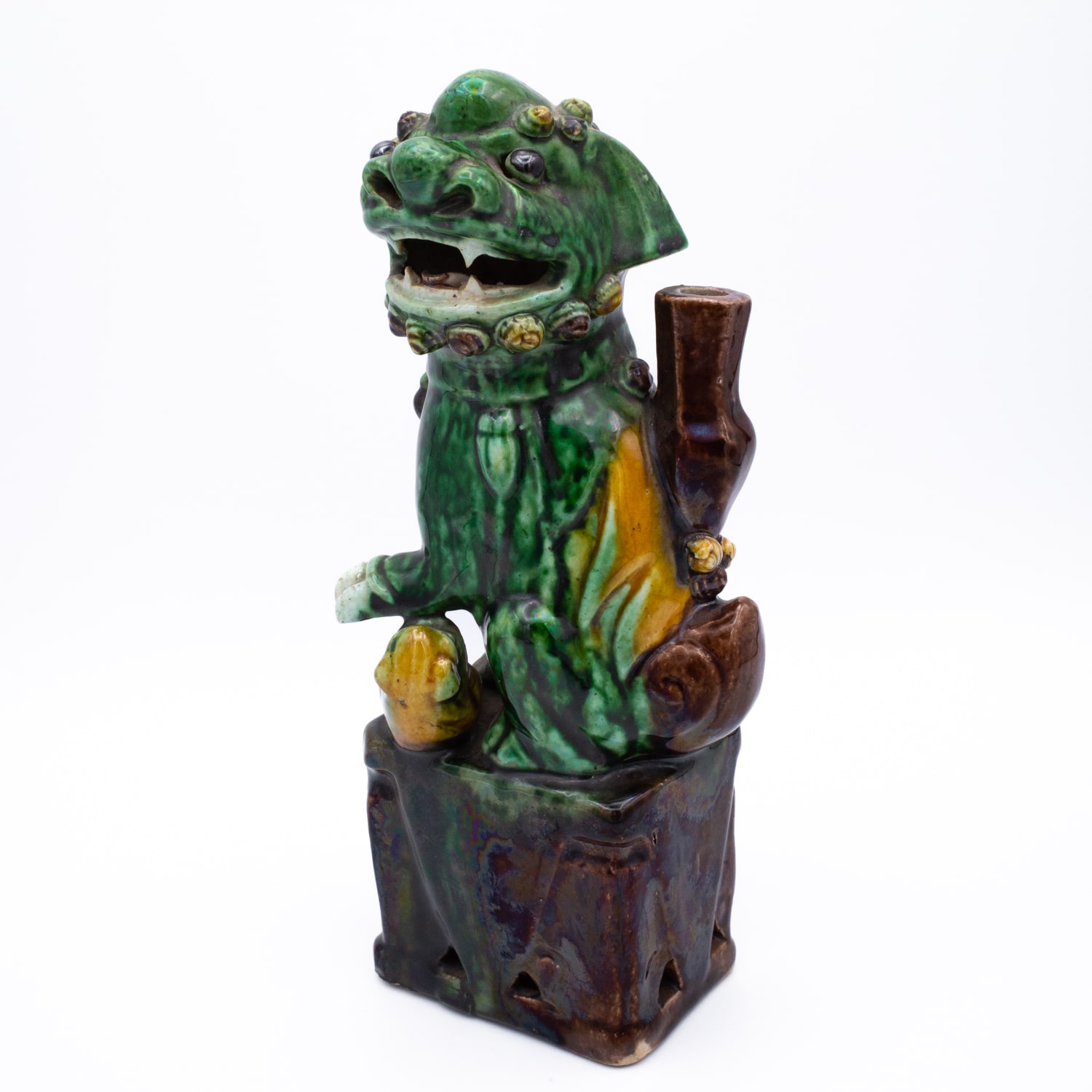This image showcases a highly detailed, decorative sculpture that merges a fantastical and somewhat mythical figure. The small statue appears to be made of a jade-colored, glossy ceramic material, giving it a shiny, finished appearance. The creature is a composite, somewhat dragon-like with canine features, characterized by its deep green paint. It has small eyes and a big, wide flared nose, and its mouth is open to reveal sharp, pointy teeth, top and bottom. The statue is adorned with intricate decorations under its chin and atop its head, adding to its ornate and possibly cultural significance.

Emerging from a wooden container, the statue extends one paw, suggesting a dynamic pose. It also sports what appears to be a gun on its back and some sort of pack, though these elements add a layer of ambiguity to the figure's identity. The creature’s small eyes, large flared nose, and sharp teeth exude an otherworldly charm, while its posture alludes to it being on alert or ready to leap. Placed on a brown square base, this piece likely reflects an Asian influence, potentially serving as a good luck charm or an ornamental item found in a home. The craftsmanship, with its carved and fired finish, highlights the figure's mystique and its blend of dragon and other animalistic traits.